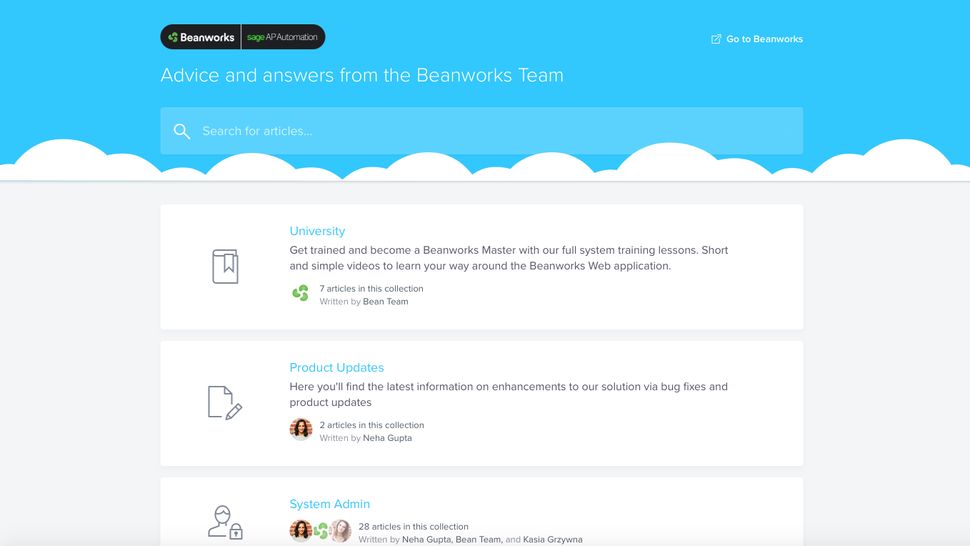The image displays the Beanworks website, which appears to be a resource hub offering articles and information on various topics, potentially enhanced with AI capabilities. The top of the page features a serene banner with clouds floating in a bright blue sky, which is visually appealing and sets a calm tone for the site. Embedded in this banner is a search bar for users to look up specific articles, accompanied by the text "Advice and answers from the Beanworks team." Additionally, there is a navigational link labeled "Go-to Beanworks" situated in the top right corner of the banner.

Below this picturesque banner, the website is organized into several clickable sections, each offering different types of content. The first section is titled "University," inviting users to "Get trained and become a Beanworks master with our full system training lessons." This section promises short and straightforward videos to help users navigate the Beanworks web application, and it contains seven articles curated by the Bean team.

The second section, "Product Updates," provides the latest information on enhancements to the Beanworks solution, including bug fixes and product updates. This section features two articles authored by Nia Gupta.

The third section is labeled "System Admin," though it lacks a descriptive introduction. Despite this, it is quite extensive, comprising 28 articles contributed by various authors. 

Overall, the website is meticulously organized to cater to users seeking training, updates, and administrative support related to the Beanworks platform.